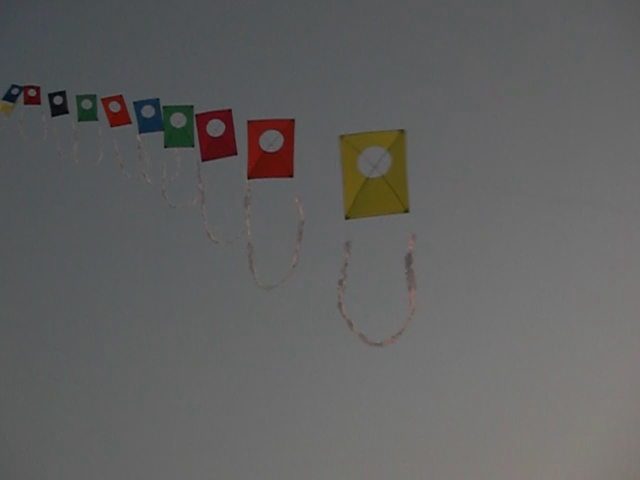A striking photograph features a line of ten colorful kites soaring against a dark, dismal gray sky, potentially due to a setting sun casting light in the upper right corner. The kites, organized in a precise linear arrangement, showcase a variety of muted colors: dark blue, red, purple, orange, blue, green, red, bright red, red, and yellow. Each kite is adorned with a distinct U-shaped draping decoration reminiscent of tinsel or a floral band, hanging from its bottom. Characteristically, every kite is a rectangle featuring a white circular section in the center intersected by an X-shaped pattern. The kites appear to get smaller as they recede into the distance, all uniformly facing the same direction, as if flown simultaneously in perfect synchrony.